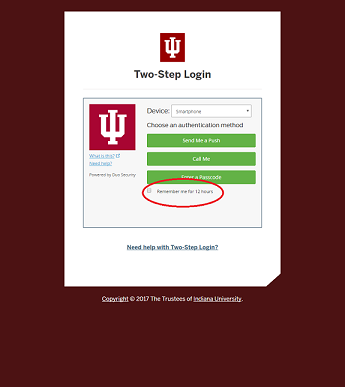The image is a partial screenshot from an Indiana University webpage, focusing on the login section. The background is predominantly burgundy, with a prominent white rectangular section in the center. The white area features the Indiana University logo, which resembles a candelabra or menorah but is actually a stylized combination of a capital 'U' and capital 'I'. Below the logo, the text "Two-Step Login" is displayed, with a drop-down menu for selecting the type of device for login—in this case, a smartphone. There are three green buttons beneath the drop-down menu, labeled "Send Me a Push," "Call Me," and "Enter a Passcode." Below these options, there is a checkbox labeled "Remember me for 12 hours," which has been circled in red to highlight its importance. This red oval emphasizes the specific focus of the screenshot, which is to draw attention to the "Remember me for 12 hours" option.